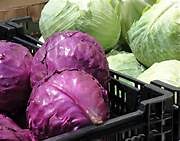The image appears to be a close-cropped, detailed shot of a grocery store display, focusing on two black crates placed side by side. The crate on the left contains vibrant, fresh, and ripe purple lettuce (mistakenly thought to be purple onions in one description), while the crate on the right holds equally fresh and ripe green lettuce, likely iceberg. Both crates are filled with large, round, and full heads of lettuce with long leaves enveloping them. The black crates seem to be positioned against a brown wooden backing or wall, which is slightly visible in the upper corner of the image. The overall scene suggests a well-stocked, visually appealing produce section in a supermarket, emphasizing the healthy and bright appearance of the lettuce heads.